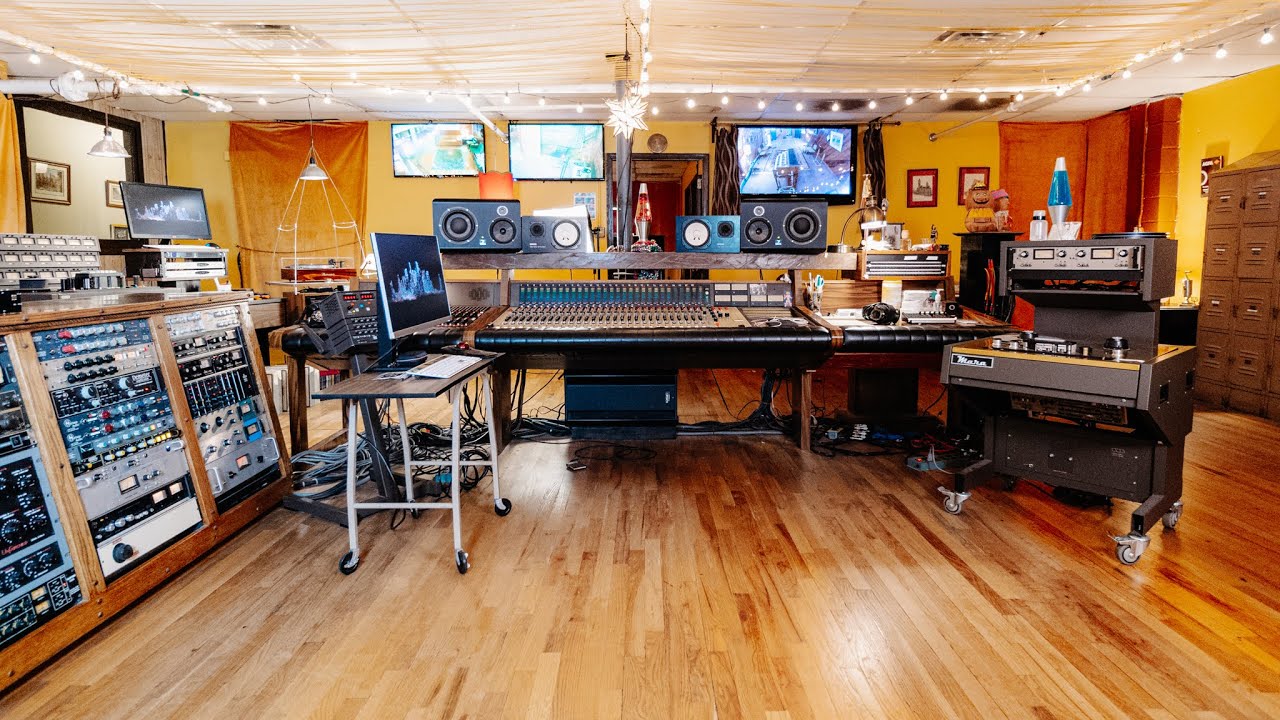The image depicts a spacious, horizontal rectangular recording studio with highly polished brown hardwood floors and golden yellow walls. The ceiling is white and adorned with string lights along the border, adding a subtle glow to the room. Centrally featured is a large console area with a sleek silver switchboard filled with numerous sliders and controls, clearly designed for musical recording. Surrounding the console are several computer monitors and television screens mounted on the wall, providing ample visual information to the operator.

On the left side of the room, a variety of equipment is visible, including a grand piano and a sophisticated rack mount built into a wooden case unit, featuring a myriad of sliders and knobs. This side also houses a wooden table on rolling wheels, supporting a monitor and keyboard, and multiple chairs. Several filing cabinets stand against the walls, contributing to the functional atmosphere of the studio.

The right side showcases additional heavy-duty machinery, possibly for vinyl cutting or similar activities. A microfiber in the middle of the room indicates it is likely used for audio recording. Numerous wires snake across the highly polished floor, connecting various pieces of equipment.

There are also two brown wooden doors: one closed on the left side and another open on the right. Pictures and framed artworks decorate the back wall and parts of the side walls, adding a touch of personal flair to this high-tech space. Various speakers are strategically placed around the room to ensure optimum sound quality. The overall setup speaks to a well-equipped recording studio, designed for both functionality and creative flexibility.